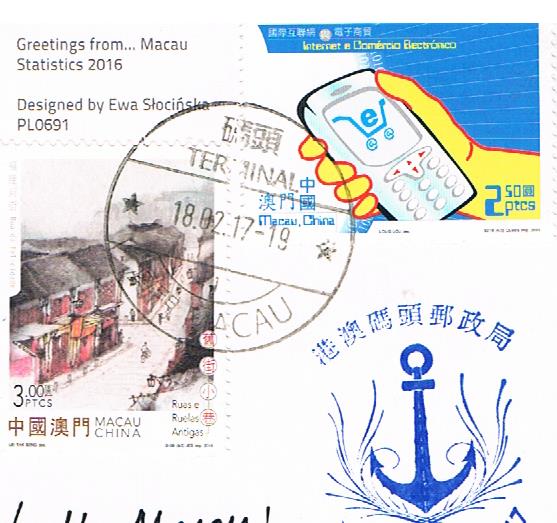This image appears to be a detailed postcard from Macau, featuring distinct elements indicative of its origin and style. At the top left corner, bold text reads "Greetings from Macau," with a subheading, "Statistics 2016," and below that, it credits the design to Iwa Słoczka, followed by "PLO 691." A prominent feature on the left side is a stamp displaying a picturesque town street in Macau, marked with "3.00" at the bottom left and "Macau, China" along the bottom. This stamp is partially overlaid by a round postmark that includes the word "Terminal," a date, and other symbols. In the top right corner of the postcard, there's an image of a yellow hand holding a cell phone with some indiscernible writing above it. In the bottom right, a blue anchor is depicted with Asiatic symbols positioned above it, accompanied by a small blue triangle in the corner. Lastly, there are fragmented letters protruding from the bottom left corner, adding a mysterious, incomplete element to the overall design.